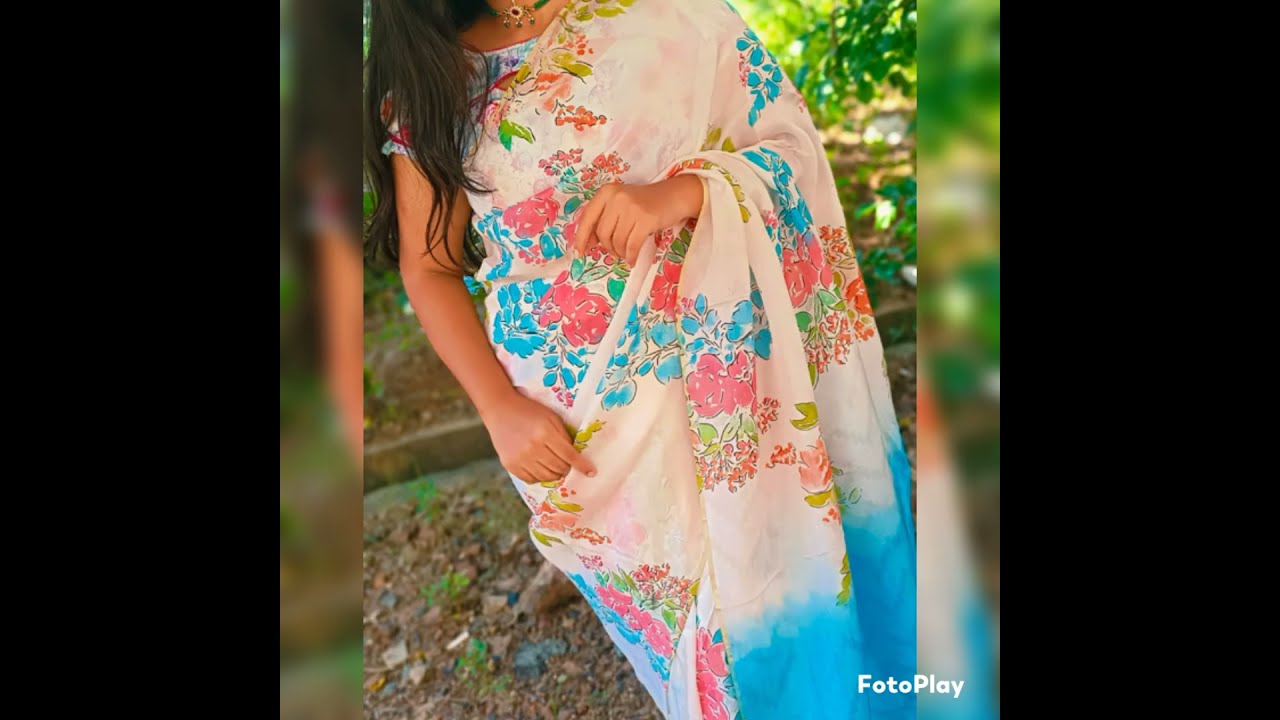The image is a horizontally rectangular photograph taken outdoors on a sunny day. It predominantly features a woman standing in a garden area, though her face is not visible as the photograph is cropped from her neck down. She has long black hair cascading down her left side. The woman is dressed in a traditional Indian sari, which is cream or white with blue and red flower designs accompanied by green leaves. The sari drapes elegantly over her left arm while her right arm remains bare. The bottom of the sari is a striking blue. The photo is bordered by wide, dark black strips on either side with narrow reflective strips adjacent to them, showing reflections of her arm and the garden surroundings. The setting is a dirt path amidst lush green foliage and illuminated by sunlight. A blue choker with a sun-shaped gem adorns her neck. The ground beneath her includes dirt, stones, and some green plants. In the lower right-hand corner, the text "PHOTO PLAY" is visible in white font.